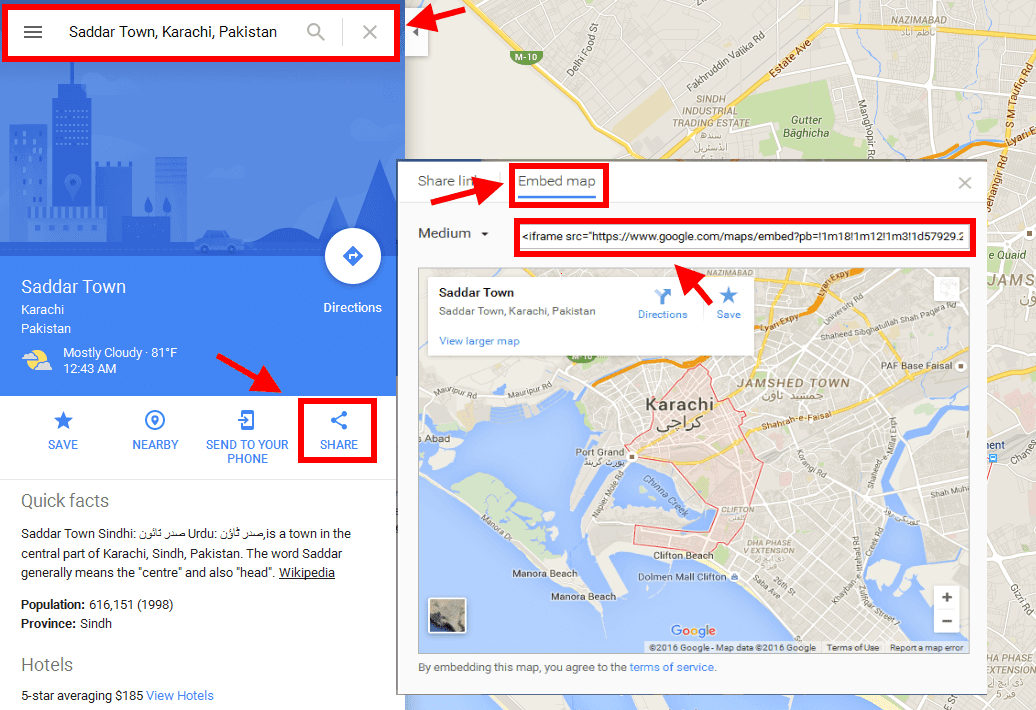A digital map interface prominently displays Sardar Town in Karachi, Sindh, Pakistan. The map highlights the current weather in Sardar Town as mostly cloudy, with a temperature of 81 degrees Fahrenheit at 12:43 AM. A quick facts section below the map offers additional details: Sardar Town is located in the central part of Karachi and primarily speaks Sindhi and Urdu. According to data from 1998, the population stands at 616,151. The word ‘Sardar’ typically signifies both 'center' and 'head,' as noted by Wikipedia. 

Adjacent to this section, a list of local accommodations shows an average five-star hotel price of $185. Nearby, an enlarged close-up view of Sardar Town, framed by a red arrow and labeled "embed map," provides a focused look at Karachi's central area. Accompanying this detailed view is a URL for Google Maps, offering a direct link to the specified location. Below the initial map window, four links provide further pages about Sardar Town, while a prominently highlighted share icon, accented in red, underscores the ease of distributing this detailed geographical and socio-cultural information.